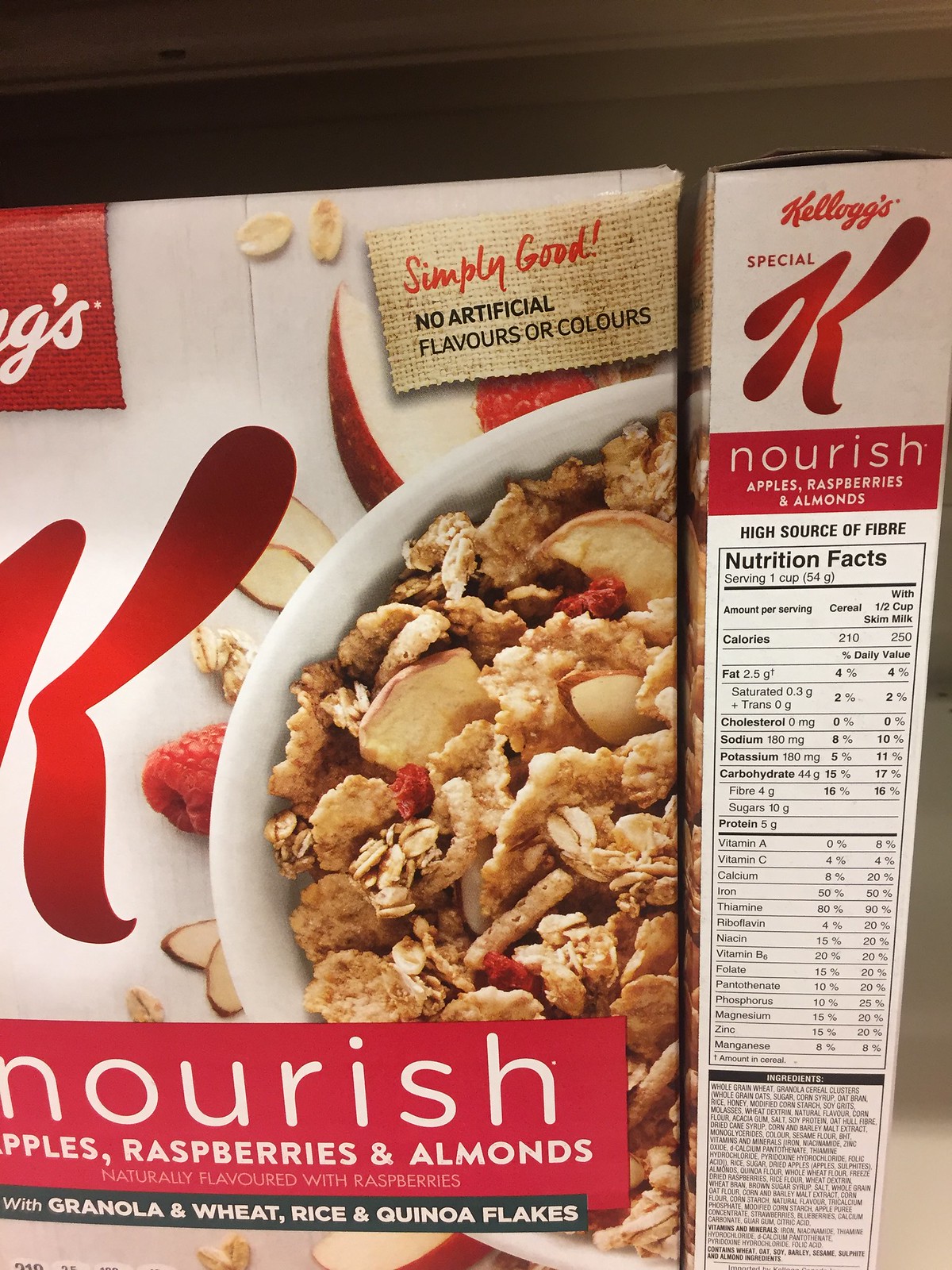The image features two boxes of Kellogg's Special K Nourish cereal prominently displayed on a white shelf against a white background. The front of one box faces the camera, showcasing the vibrant design elements and text, while the other box is positioned to reveal its side, showing the detailed nutrition facts and ingredients list.

The front of the box is predominantly white with striking red and pink accents. The iconic Kellogg's Special K logo in bold red cursive is prominently displayed. Below the logo, there's a burlap label in the top right corner stating "Simply Good - No Artificial Flavours or Colours," with the British/Canadian spelling of "flavours" and "colours." This indicates it's a version possibly marketed outside the United States.

Beneath this label, a white bowl overflowing with the featured cereal is depicted, containing apple slices, raspberries, and almonds, which are also artistically arranged around the bowl. The descriptive text on the front emphasizes "Nourish Apples, Raspberries, and Almonds," along with smaller text detailing that it's "Naturally Flavored with Raspberries" and includes "Granola and Wheat, Rice, and Quinoa Flakes."

The side of the box visible in the image provides a closer look at the nutritional information and the ingredients list, which are printed in small, fine text. The detailed and colorful design elements perfectly encapsulate the nutritious and appealing nature of the cereal.